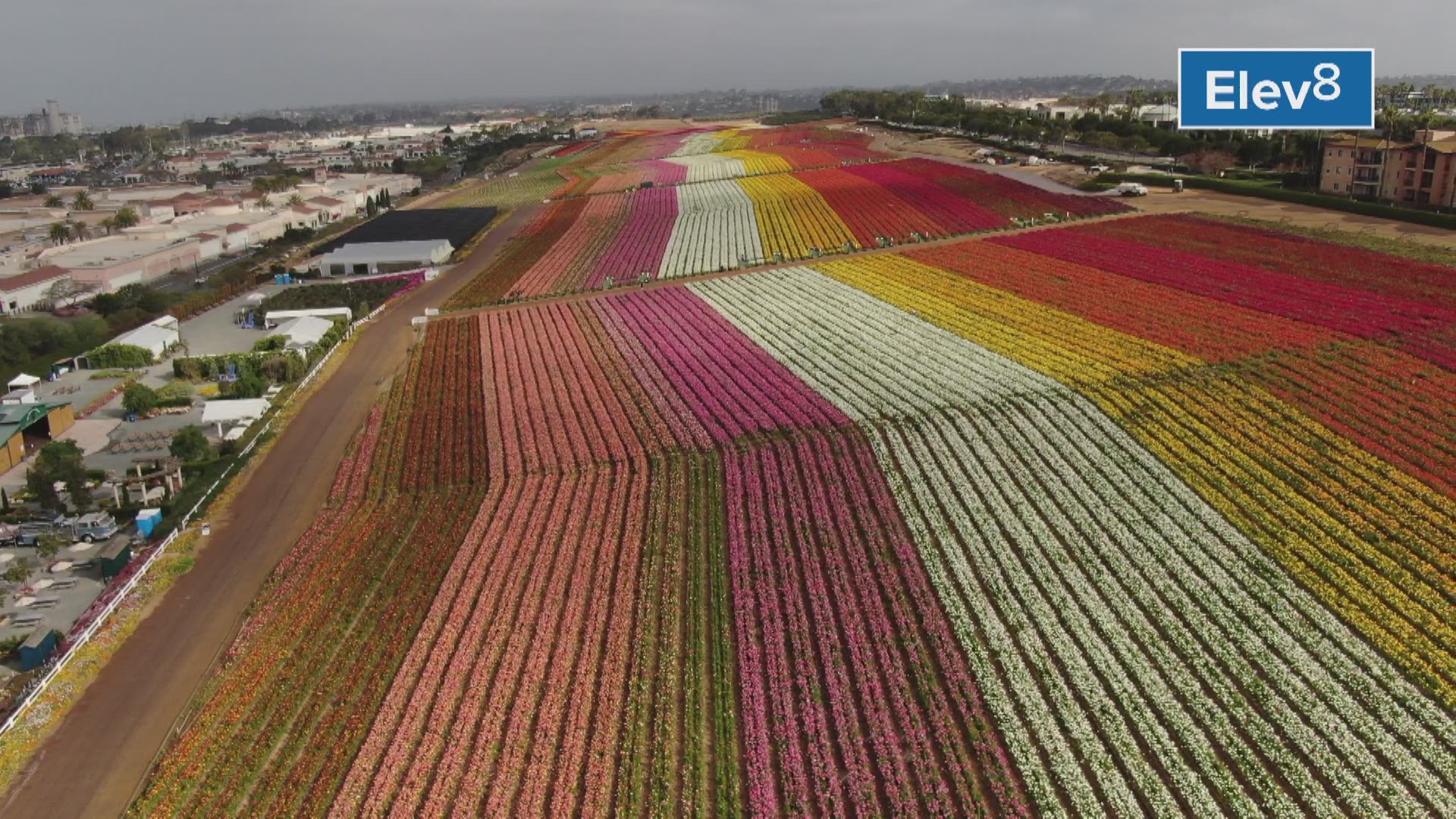This vibrant landscape photograph showcases a meticulously cultivated stretch of land, nestled between industrial and residential areas, characterized by orderly rows of blooming flowers. The scene is vividly colorful, featuring stripes of flowers in a spectrum of hues. Starting on the left, the field displays green, light pink, and lavender pink, transitioning through shades of amethyst, white, light yellow, dark yellow, orange, bright fuchsia red, to darker red, possibly a variety of mums given their recognizable colors. The stripes extend far into the distance, adding depth to the image. The fields are bordered by roads on either side, with an array of buildings scattered around, emphasizing the striking contrast between the lush floral landscape and the surrounding built-up areas. A label marked "ELEV 8" is seen on one side of the field, adding a quirky detail to this unusually colorful agricultural scene amidst urban surroundings.